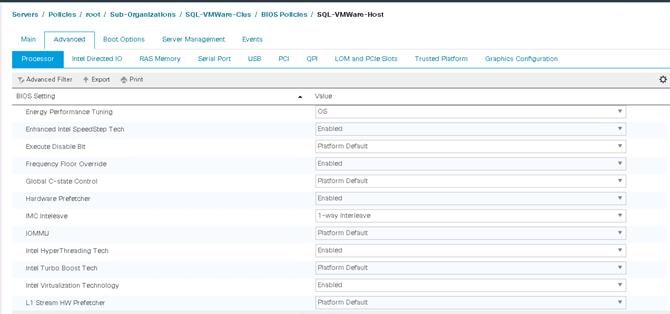### Detailed Descriptive Caption:

This image is a screenshot of the SQL_VMware_host settings page within a management interface. At the top of the screen, a breadcrumb navigation bar details the path to this particular page, starting from 'service policies' and traversing through 'root', 'sub-organizations', 'SQLVMware', 'BIOS', and 'BIOS policies', ultimately reaching the 'SQLVMware/host' page.

Below the breadcrumb, there is a series of main tabs including 'Main', 'Advanced', 'Boot Options', 'Server Management', and 'Events'. The screenshot specifically shows the 'Advanced' tab selected and active.

Within the 'Advanced' tab, multiple configuration categories are listed, including 'Policy', 'Barrage Memory', 'Serial Port', 'USB', 'PCI', 'Trusted Platforms', and 'Graphic Configuration'. Each category likely contains various settings and options related to the advanced configurations of the VMware host. The settings are displayed in a tabular format, with data organized into left and right columns for easy navigation and comparison.